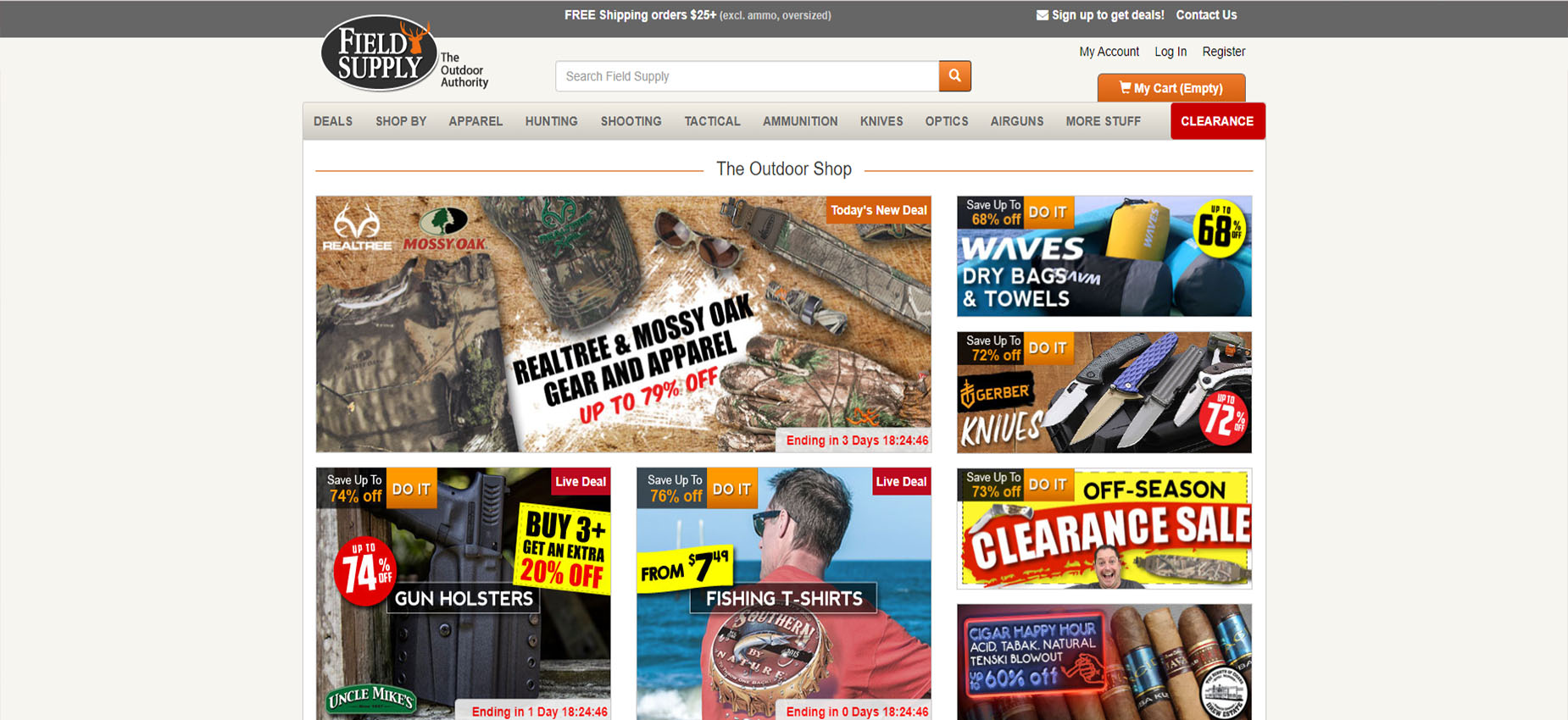Here is a detailed and cleaned-up caption:

"The Field Supply website is prominently displayed, featuring its distinctive logo with the words 'Field Supply' accompanied by an orange deer's head and antlers. Branded as 'The Outdoor Authority,' this site caters to enthusiasts looking for outdoor gear. The main webpage showcases various deals prominently at the bottom, including fishing t-shirts starting at $7.49 and a clearance sale offering up to 72% off on off-season knives. Images of current sale items enhance the shopping experience.

At the top, several categories are available to help users narrow their search, including Apparel, Hunting, Shooting, Tactical, Ammunition, Knives, Optics, Air Guns, and more. There's also a dedicated tab for clearance items. In the upper right-hand corner, users can log in or register for an account, and there is a cart icon where shoppers can view their selected items."